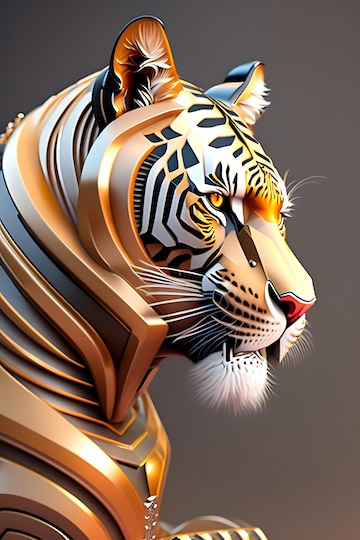The image depicts a three-dimensional rendering of a tiger with a visually compelling, almost sculpture-like appearance. The tiger is presented in vibrant, sharp hues of orange, white, and black. It has striking orange eyes and a bright red nose tip, adding vivid detail to its face. The tiger appears to be made of plastic or metallic bars, giving it an armored look rather than natural fur. This 3D-rendered figure shows only the front part of the tiger, including its head, chest, and part of one paw with visible claws. The tiger's ears are orange with a hint of black, complementing its white-striped face. The creature looks to the right, set against a predominantly dark, blackish-brown background, giving it a poised and contemplative appearance, as if observing something intently.